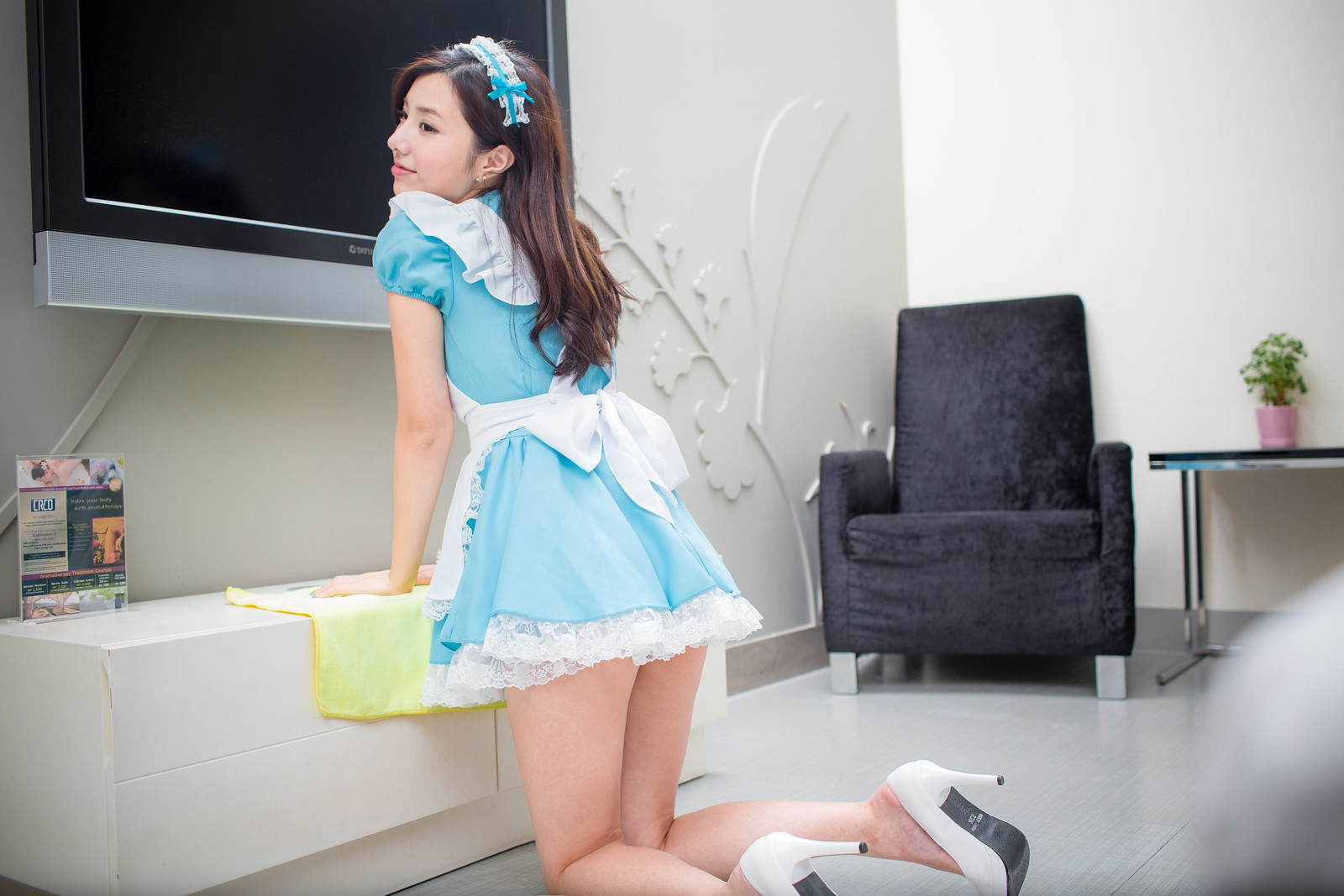In the image, a young woman with long, dark brown hair is wearing a sky blue dress reminiscent of Alice in Wonderland. The dress features poofy sleeves, a white trim, a lace apron, and a short, fluffy skirt adorned with white lace at the bottom, complemented by a lacy blue and white headband. She is on her knees, delicately placing her hands on a white TV stand, with a yellow towel underneath her, as she looks over her shoulder and smiles. 

The woman is also wearing white high heels and appears to be in a bright, impeccably clean setting with predominantly white walls and floors. A large TV is mounted above the TV stand, and to the side, there's a black, comfortable chair with silver legs, and a small table beside it adorned with a green plant in a pink vase. The image seems to depict a polished environment, possibly indicative of a business or a hotel space rather than a typical home, suggested by the presence of an advertisement on the console table.